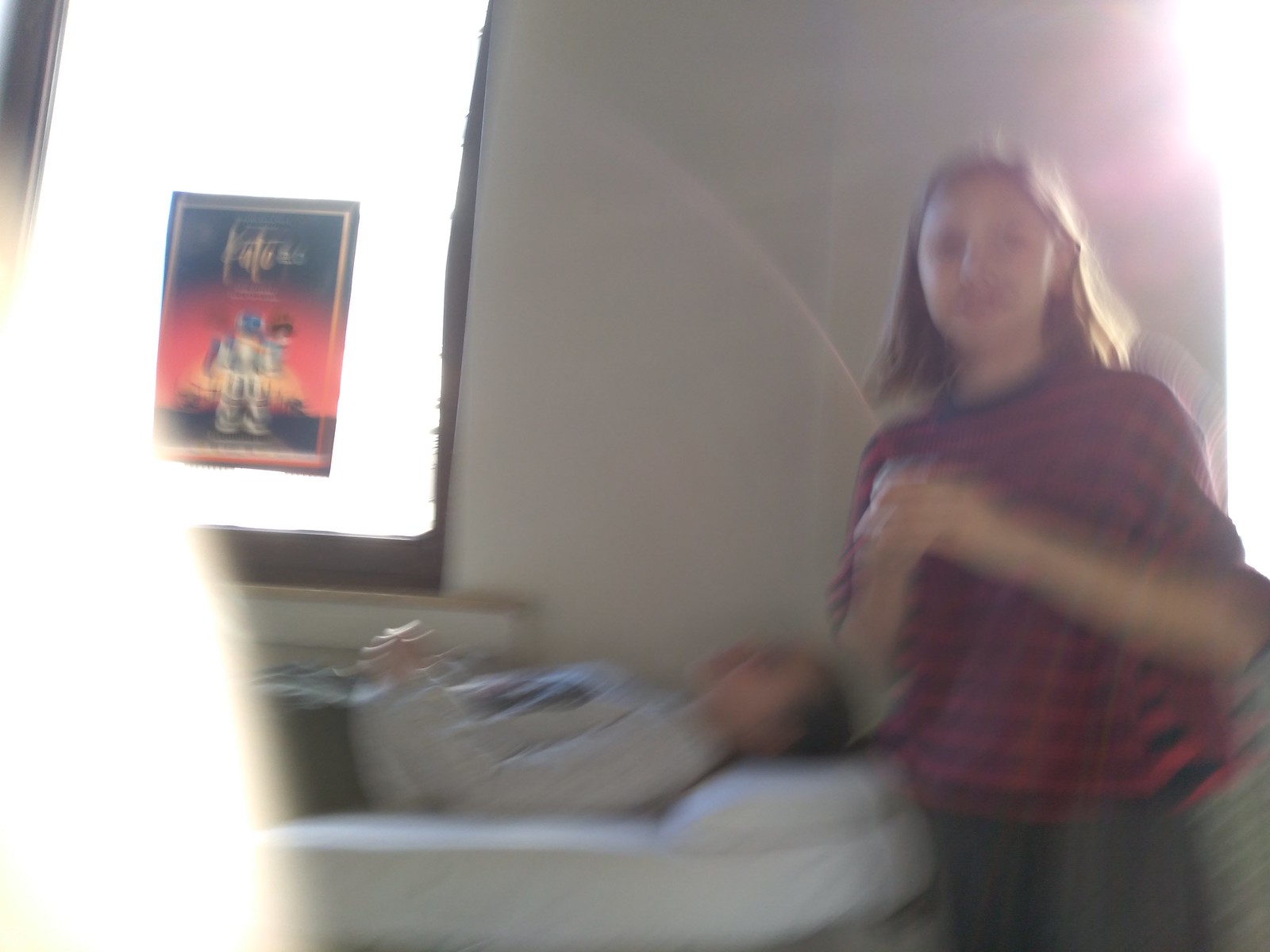In a somewhat blurry photograph, the interior of a room is depicted with notable elements that catch the eye. On the right side of the image, there is a young person with shoulder-length dark brown hair. They are dressed in a short-sleeved, red and black striped shirt paired with gray pants. Centrally positioned in the image is another individual who appears to be lying on their back, very still, with hands crossed over their stomach. This person might be asleep or possibly deceased, contributing to an eerie stillness. They are on a white mattress with a matching white pillow, facing upward toward the ceiling. They are dressed in a long-sleeved gray shirt and dark gray pants, sporting short, possibly grayish or dark hair.

Toward the left, there is a window adorned with a poster that seems to advertise a TV show or movie featuring a robot character. Despite the overall blurriness of the photo, these details emerge, giving a glimpse into the room's unsettling atmosphere and the enigmatic presence of its occupants.